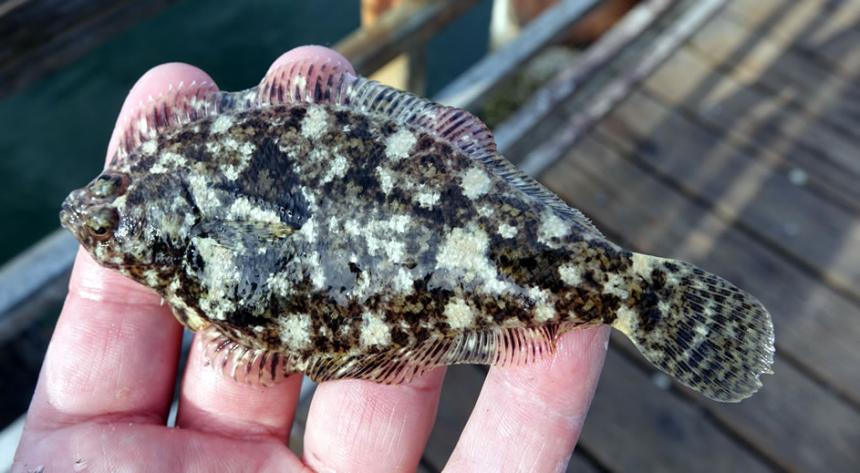This is an image of someone holding a small, flat fish that appears to be a baby flounder. The fish is resting across the top four fingers of the person's left hand, which has pale skin and short, stout fingers. The fish itself is about the length of these four fingers and features a mottled pattern of olive green, tan, black, brown, and cream-colored speckles. Its eyes are both on the same side of its head, and it has small, beady black eyes near slits that resemble gills. The fish has continuous fins running along the top and bottom of its flat, pancake-like body, and its tail is rounded. In the background, slightly blurred, is a wooden pier or dock with metal railings and a glimpse of the water on the left, along with shadows indicating it is a sunny day. The close-up nature of the photo focuses on the fish and the hand, highlighting the fish's unique and camouflaged appearance.